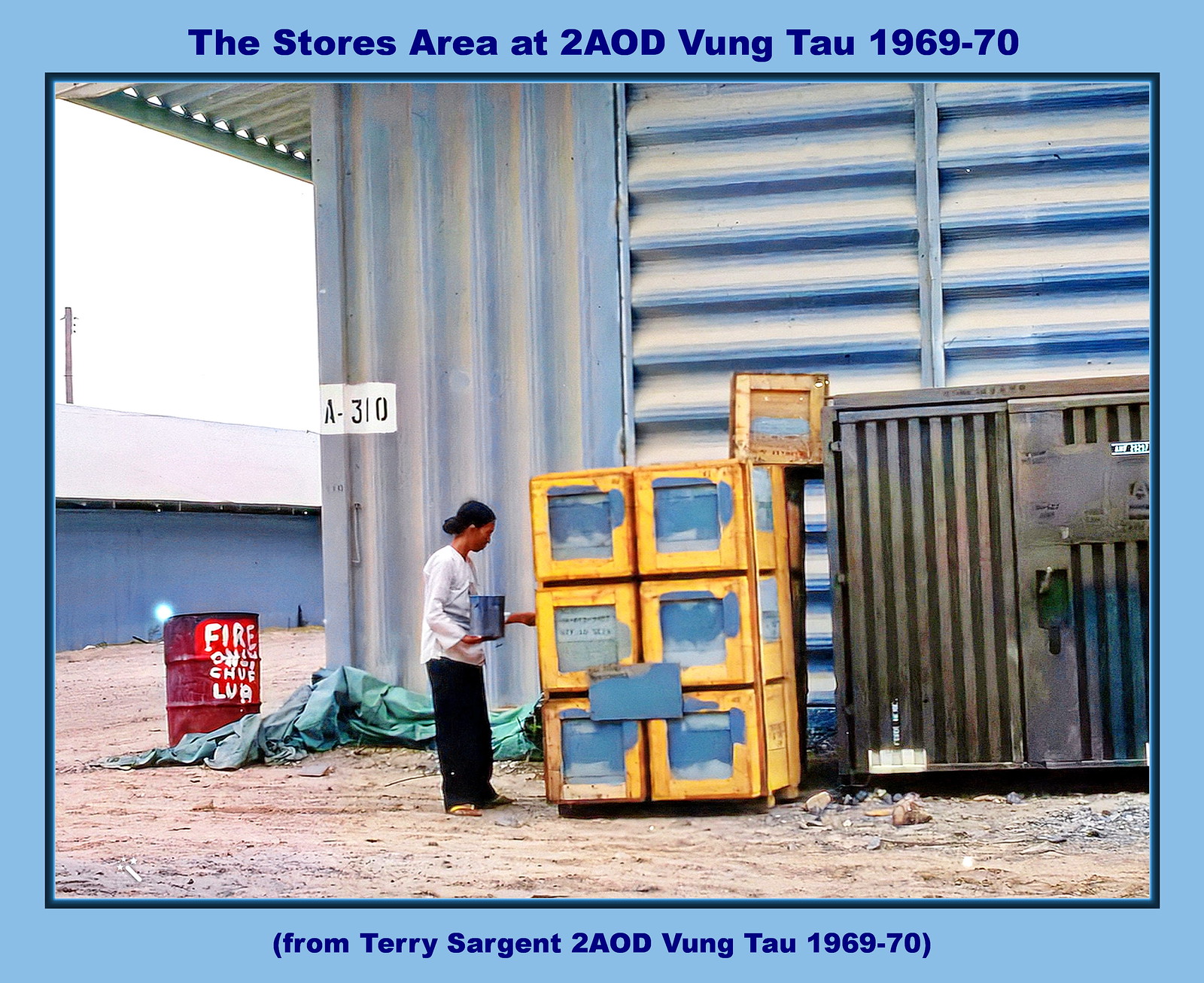The postcard image, bordered by a light blue trim and darker blue inner frame, captures an outdoor scene set against a large industrial tin building. This structure, with its sheet metal walls and roof, features a column of vents on the right side and a white box labeled "A-310" halfway up the left side. The photograph, dated 1969-70, and attributed to Terry Sargent, is from "The Store's Area at 2 A.O.D. Vung Tau."

In the center of the image stands a woman with dark hair pulled into a bun, wearing a white blouse and black pants. She is focused on a yellow palette or series of six yellow cubes, appearing to place a blue box into one of them. Nearby, a red oil drum marked "fire" is connected to the yellow cubes by a green tarp. The surrounding ground is a dirt and sand mixture, suggesting an outdoor setting despite some indoor elements like a large metal dumpster or locker to the right. Additional features include a palette of yellow boxes with blue paint splashes and a red bucket labeled by hand. The overall color scheme of the scene is dominated by blues and grays.